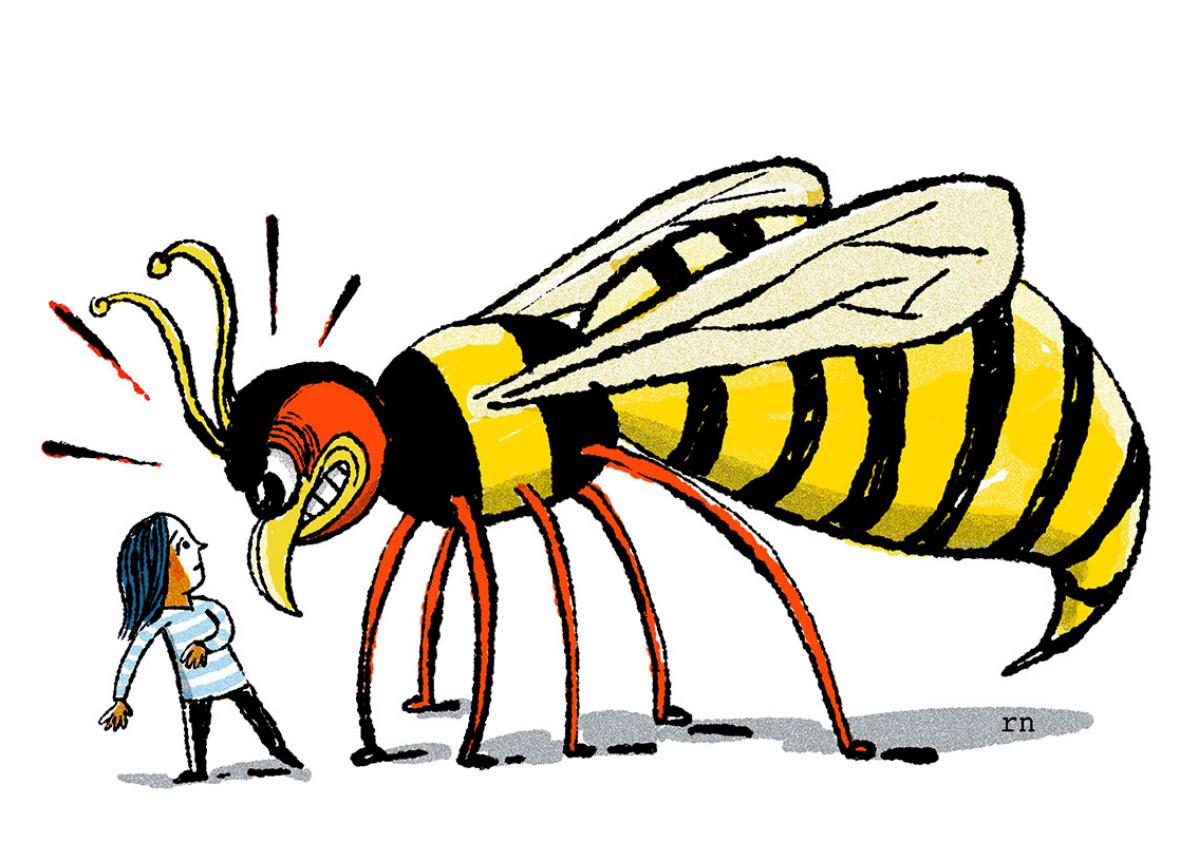The image is a detailed cartoon drawing featuring an oversized wasp or bee and a small girl, both depicted in vibrant colors against a stark white background. The wasp has a black and yellow-striped body with a large, ominous stinger, complemented by off-white wings and red-orange legs. Its red face, adorned with a white beak and yellow antennae, is locked in an angry grimace as it peers directly at the girl. The girl, shown in profile, is wearing a long-sleeved, light blue and white striped shirt with black pants. Her blue, shoulder-length hair frames a fearful expression as she stares back at the towering insect. The scene is accentuated by the shadows cast by both characters, and the text "R.N." is subtly placed in the bottom right corner of the image, adding a final touch to the striking composition.